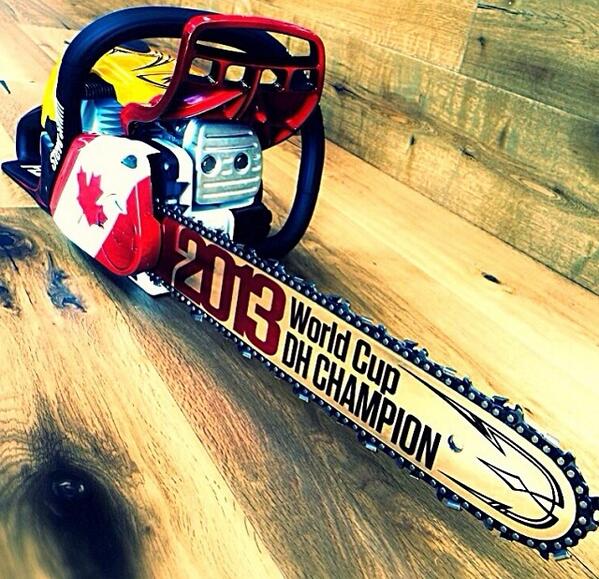The image depicts a chainsaw resting on a light brown wooden table, which features noticeable black knots and darker stains. The chainsaw itself is a vibrant mix of colors: the motor housing is painted yellow, while the handle is a striking blue with some red detailing. The side of the chainsaw showcases a design resembling the Canadian flag, with a prominent red maple leaf set against a white background framed by red. The blade, bordered by a black chain link, bears the inscription "2013 World Cup DH champion" in maroon and black lettering, with a decorative pinstripe accentuating the top curve. The scene is illuminated by subtle light, emphasizing both the tool’s celebratory markings and the textured surface of the wooden tabletop.